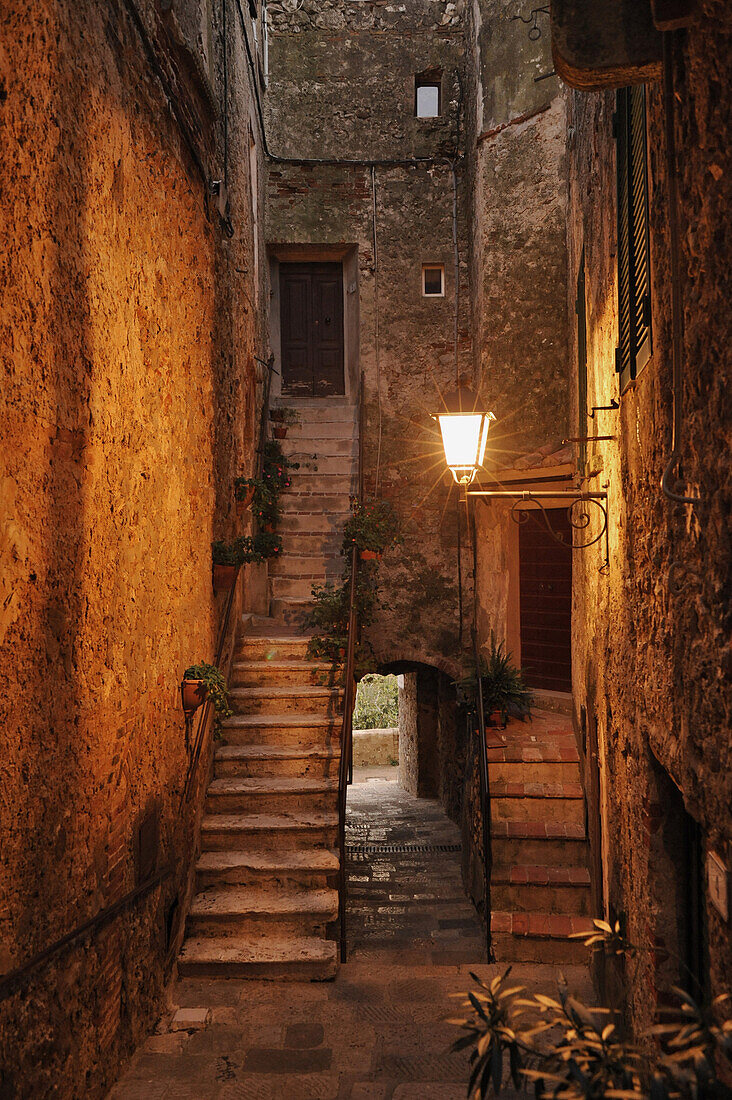The image depicts an old stone building, characterized by its weathered, brownish-gray textured walls. On the left side of the vertically aligned rectangular image, a stone wall runs from top to bottom. Adjacent to this wall, a narrow staircase with approximately twelve cement steps ascends to a wooden door. This stairway features small potted plants and guard rails along its sides. Above the wooden door, the aged grayish-brown stone wall shows two rectangular cutouts. 

In the middle of the image, to the right of the stairs, there is a covered, arched walkway that seems to lead outside, where trees are visible. Further to the right, stone tiles form another set of stairs leading up to another flat area with a door. This second stairway is possibly part of a small alleyway and includes additional greenery near the bottom of the image. A light fixture hangs in the middle of the scene, illuminating the area and adding to the ambiance of an old village-like setting, potentially in a foreign country such as Italy.